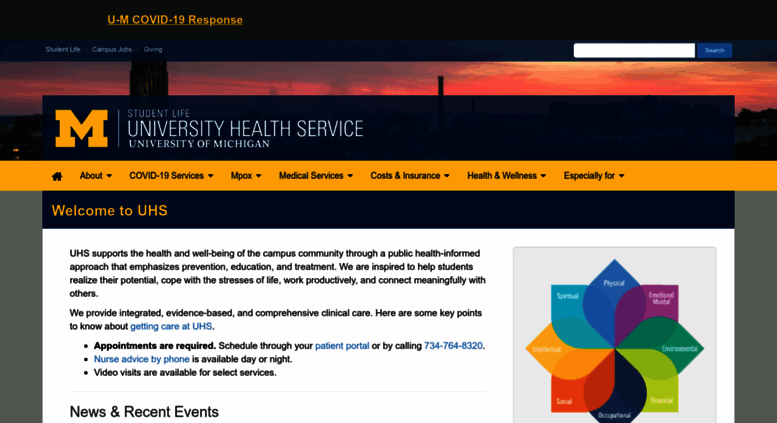Landscape-oriented and slightly wider than tall, this image appears to be a press release or homepage feature from the University of Michigan website. At its top, a dark gray border features yellow, underlined text that reads "U-M COVID-19 Response." Below this is a semi-transparent dark blue bar where the background is faintly visible. On the left side of this bar, in white text, are links labeled "Student Life," "Campus Jobs," and "Giving." On the right, a white search bar accompanied by a blue and white search button sits prominently.

The background image captures a cityscape at sunset, likely representing the University of Michigan campus. Overlaid on this backdrop is another semi-transparent blue box. On the left of this box is a prominent yellow "M," while to its right are white text labels: "Student Life," "University of Health Services," and "University of Michigan."

Beneath this, a long, rectangular yellow box contains black font and several drop-down menus. Starting with a home icon, the menus are labeled "About COVID-19," "Services," "MPOCS," "Medical Services," "Cost & Insurance," "Health & Wellness," and "Especially For."

Near the bottom, bold text states "Welcome to UHS," followed by a white box housing a graph, chart, and some explanatory text, most likely pertaining to COVID-related information.